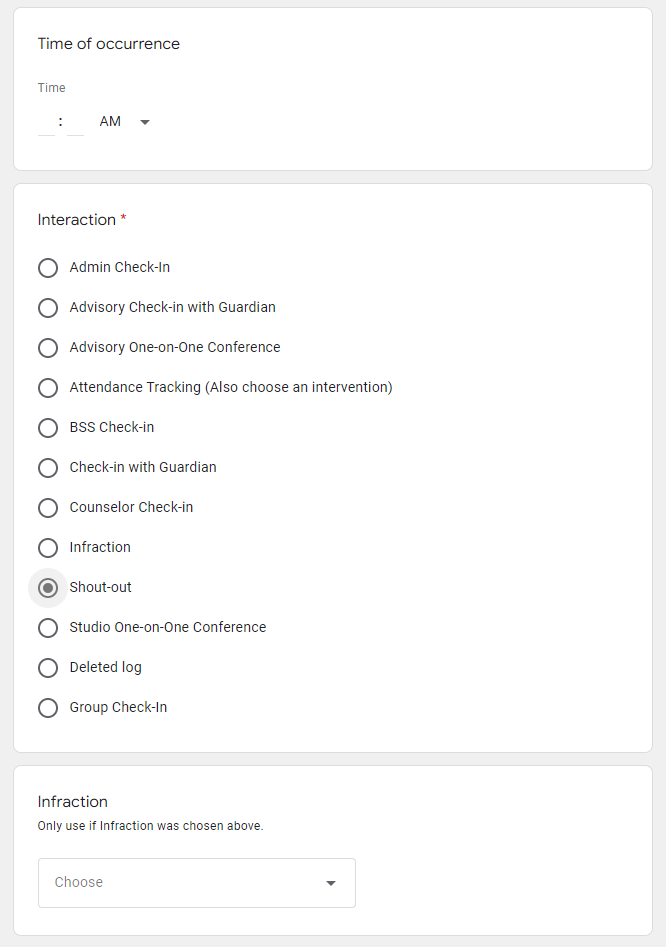The image depicts a digital form designed for recording interactions, possibly in a summer camp or daycare setting. The form features several sections, including "Time of Occurrence," where users can input the exact time of an event. Another section titled "Interaction" offers multiple options for categorizing the nature of the interaction, such as "Admin Check-In," "Advisory Check-In," "Check-In with Guardian," "Counselor Check-In," and "Infraction." In this particular instance, "Shout Out" has been selected from these choices. If "Infraction" is chosen, an additional dropdown menu appears to specify the reason for the infraction. The form is a simple, no-frills digital document, similar to those created using Google Forms, designed to facilitate the logging of various interactions and check-ins. It's utilitarian and straightforward, reflecting its purpose of streamlining record-keeping processes in an organized setting.